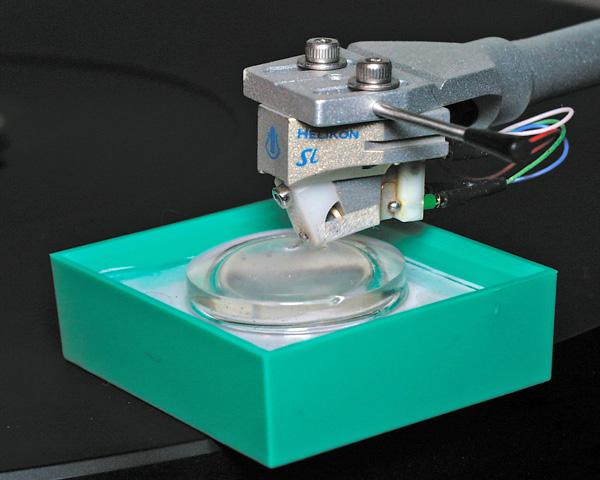This detailed, indoor, full-color photograph, taken under artificial light, showcases a close-up view of what appears to be an industrial record player arm in the production stage. The image is square without a definitive border, featuring primarily a black background. In the bottom right, there’s a solid black area, and in the bottom left, a thin gray strip extends upwards at an angle, passing beneath a light green, lidless box centrally positioned in the image. 

Emerging from the upper right corner is a prominent silver piece of electronic equipment. This apparatus, which may be part of the record player’s arm, is adorned with two silver knobs on the far left side. A notable element of this equipment is a silver lever, tipped with black rubber, extending outward. Additionally, white, blue, and green wires are visible, emanating from this device.

The green box beneath features the brand name "Heron SL" on its base. Inside the box lies a circular, clear substance, reminiscent of liquid or gel, with a glass-like object atop it. This central object—possibly the stylus or needle of the presumed record player—resembles a saucer and is partially surrounded by the liquid. Positioned just above this glass component, the apparatus includes a lighter gray piece and a white plastic part, hinting at a complex assembly process.

Completing the scene, a curve in the black background on the top left forms a subtle border, with an indented circle shape contrasting the lighter black area below it. This intricately staged photo captures the minutiae of the record player's components, emphasizing the mechanical and potentially delicate nature of its assembly.